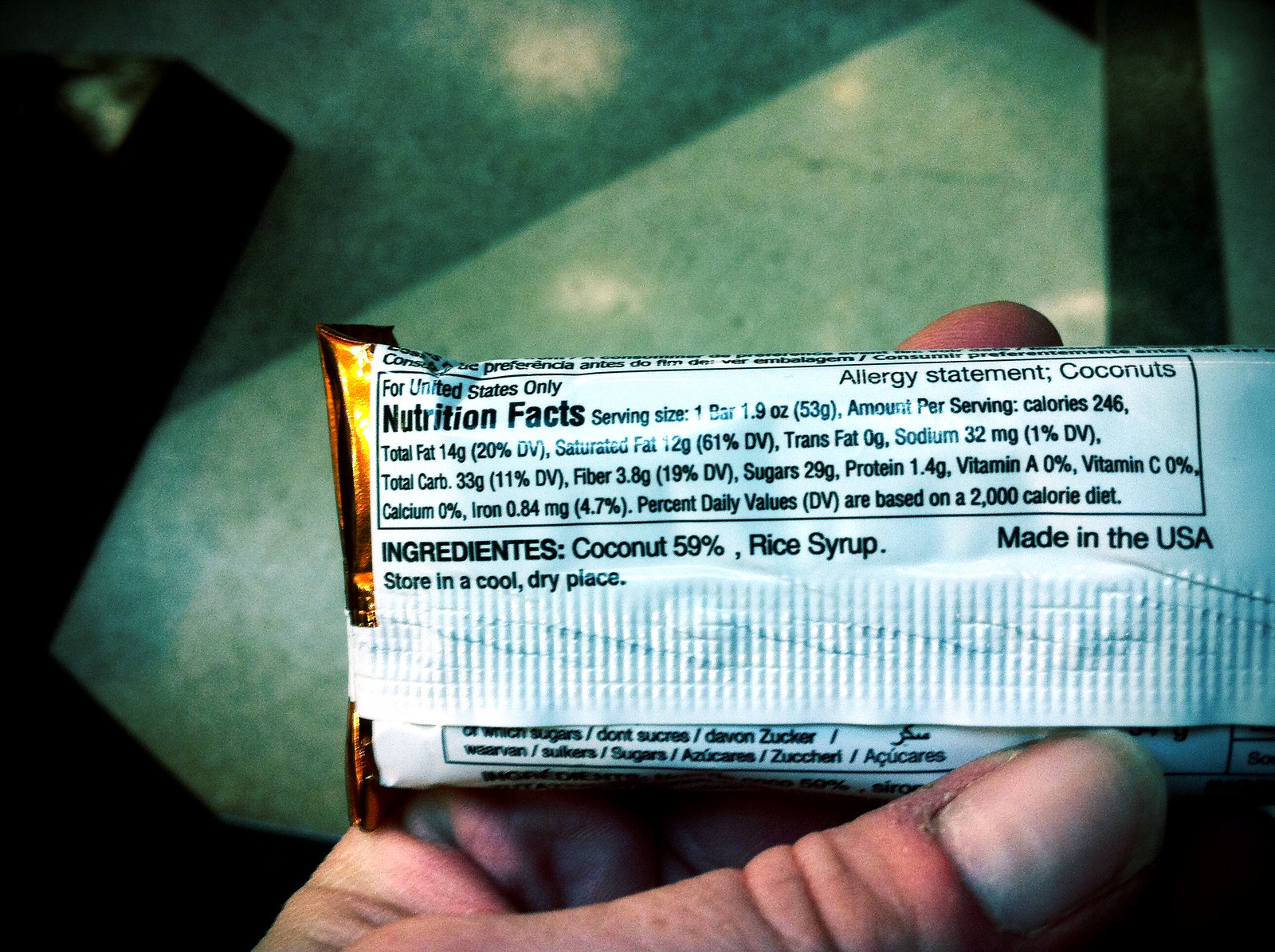The photograph features a hand holding a packaged bar against a background that appears to be a light teal-colored counter, with some black areas that are slightly blurred. The hand is positioned to show a clear view of the packaging, and upon closer inspection, the thumbnail on the left hand appears to have some dirt underneath and cracks along the edge of the nail. The bar's packaging predominantly consists of a white background with a hint of gold visible on one end. 

The text on the packaging reads:

"For United States only. Allergy statement: contains coconuts. 

Nutrition facts: 
- Serving size: one bar (1.9 ounces, 53 grams)
- Amount per serving: 246 calories
- Total fat: 14 grams
  - Saturated fat: 12 grams
  - Trans fat: 0 grams
- Sodium: 32 milligrams
- Total carbs: 33 grams
  - Dietary fiber: 3.8 grams
  - Sugars: 29 grams
- Protein: 1.4 grams

Ingredients: coconut (59%), rice syrup. Store in a cool, dry place. Made in the USA."